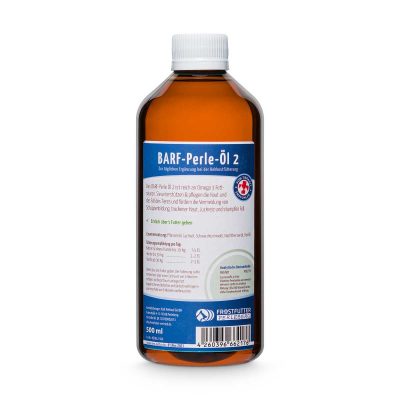The image features a brown medicine bottle, centrally positioned in a normal standing orientation with its white cap on top. The bottle has a blue and white label, with the blue section at the top bearing the text "BARF-PERLE-01C." The middle part of the label is white, adorned with small red and green writing, including a red cross inside a circle, indicative of medical use. Additional text appears in black and other white sections of the label, and a barcode is located at the bottom right corner of the bottle. The background suggests a digitally created or software-rendered advertisement focused solely on the bottle, viewed from the back.